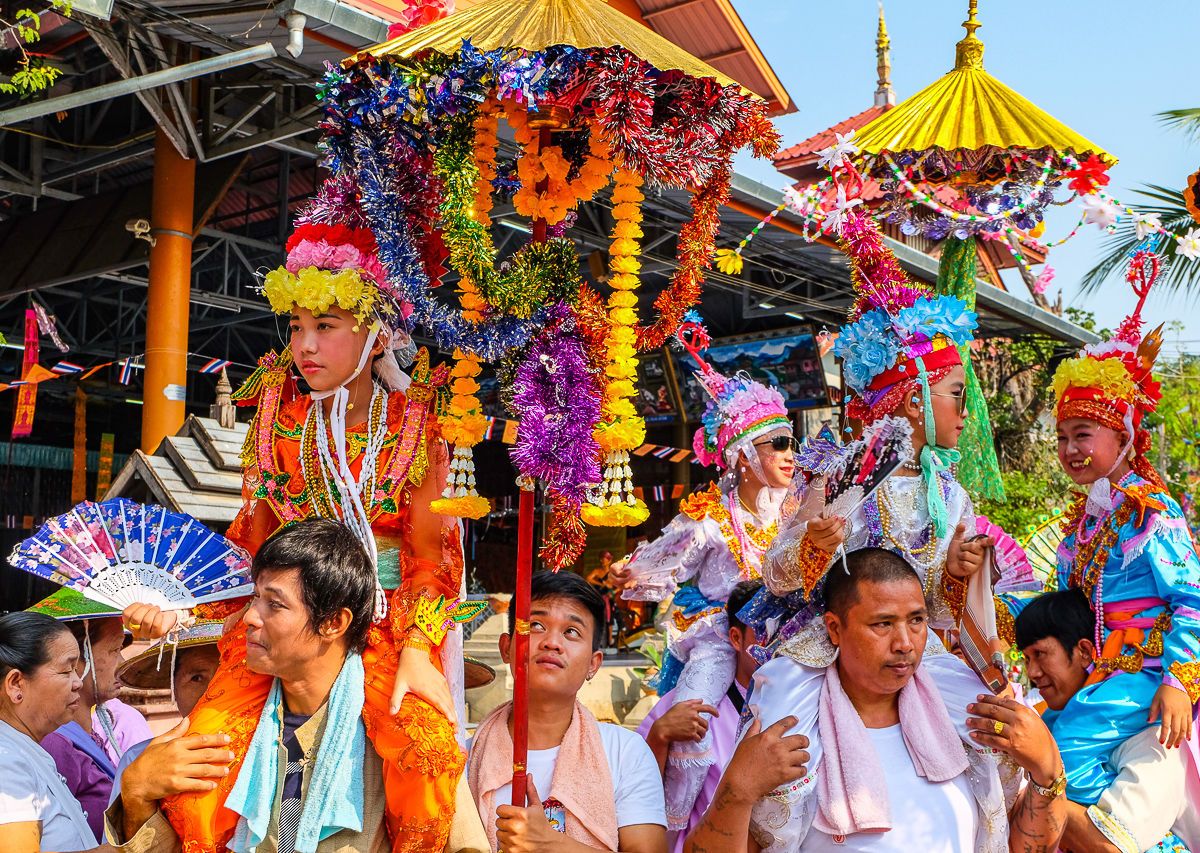This vibrant outdoor photograph, taken during the daytime, features a lively Asian cultural festival filled with vibrant colors and joyous celebration. In the foreground, four men of Asian descent are each carrying young girls on their shoulders. The girls are adorned in elaborate, colorful costumes with ornate headpieces decorated with flowers, beads, and other embellishments. Notably, one girl on the left is wearing a bright orange outfit accented with flowers and holds a blue fan. Behind the men, others hold tall red poles topped with yellow umbrellas from which garlands and flowered leis are suspended.

In the background, a covered metal structure with orange columns and exposed framework is visible, hinting at an outdoor amphitheater or stage setting. The sky in the upper right corner is a vivid blue, adding to the image's cheerful ambiance. The rich palette of yellow, green, blue, pink, and orange underscores the festive atmosphere, suggesting a celebration infused with cultural significance, perhaps Filipino or Vietnamese. The numerous decorative items, reminiscent of Hawaiian leis, contribute to the ceremonial and cultural essence of the scene.